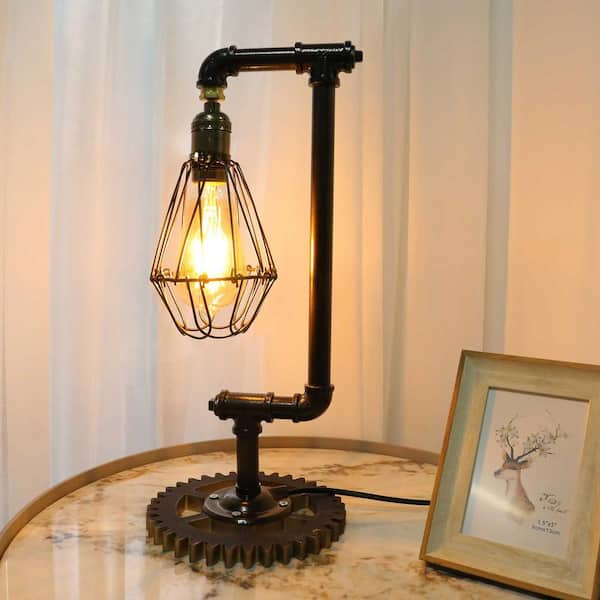The image features a unique steampunk-style lamp positioned on a round marble table with a beige and black marbled pattern. The lamp's base resembles a large metal gear, and its stand is constructed from black metal piping that forms an open U-shape. At the top of the U-shape, the bulb, an Edison-style light bulb with visible filaments, is surrounded by a black metal cage. The lamp has a black cord extending off to the right side of the image. Behind the lamp, there are white curtains, adding a lighter backdrop to the scene. In the bottom right corner of the picture, there is a small beige frame containing an illustration of a deer with leaves in its antlers and some unreadable writing on the right side of the illustration.